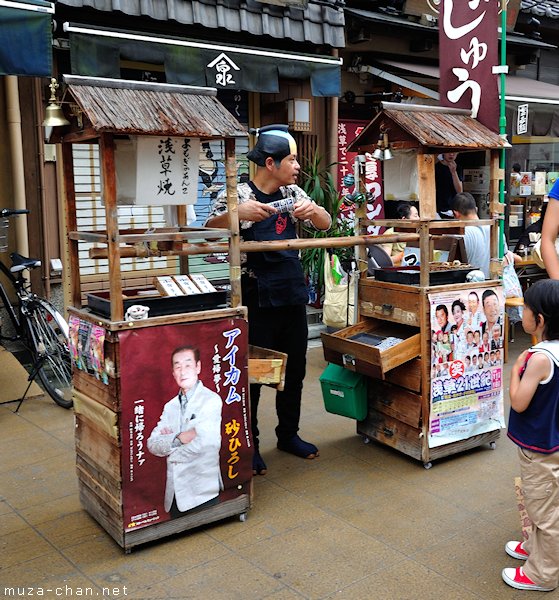The photograph captures an outdoor street vendor in an Asian market, possibly in China or Japan. The vendor is standing between two kiosks, each resembling old-style wishing wells with vaulted roofs constructed from scrap wood. The kiosks have trays on top displaying his wares, and on the front, there are posters with Asian characters advertising various products; one features a doctor in a white jacket and the other displays multiple faces. The vendor, who appears to be of Asian ethnicity, is dressed in black pants, a black apron, and a cap painted to look like a samurai helmet, with black, yellow, and green colors.

A small child, looking curiously at the vendor, stands in front of the kiosks. The child is dressed in a navy blue shirt, khaki pants, red and white sneakers, and a sailor hat. In the background, there are shops with awnings and Asian script, as well as a black bicycle parked nearby. The lower left-hand corner of the photo features the website address musa-chan.net. The entire image is presented in a rectangular frame.